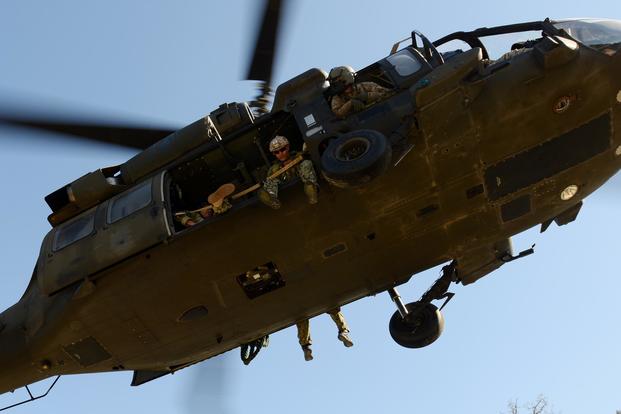The photograph captures a dramatic upward perspective of a large military helicopter, possibly a Blackhawk, against a backdrop of a clear, cloudless blue sky. The helicopter is predominantly a dark olive green with a rustic tint, and the blades are visibly mid-spin, with two distinctive blades noticeable in the top left of the image.

In the center of the frame, a soldier in dark green to gray camouflaged uniform and helmet sits at the open side door, his feet dangling freely below. Another foot extends out to the left side, obscured by the helicopter's structure, suggesting the presence of another soldier. To the right, a third military personnel peers back from the passenger side window, similarly dressed in combat uniform and helmet, adding to the sense of action and gravity.

Towards the bottom half of the image, more legs are seen dangling from the opposite side, near the underbelly of the helicopter, accompanied by a glimpse of the landing gear wheel. The entire composition showcases the rugged readiness of military activity, framed by the contrasting serene blue sky.